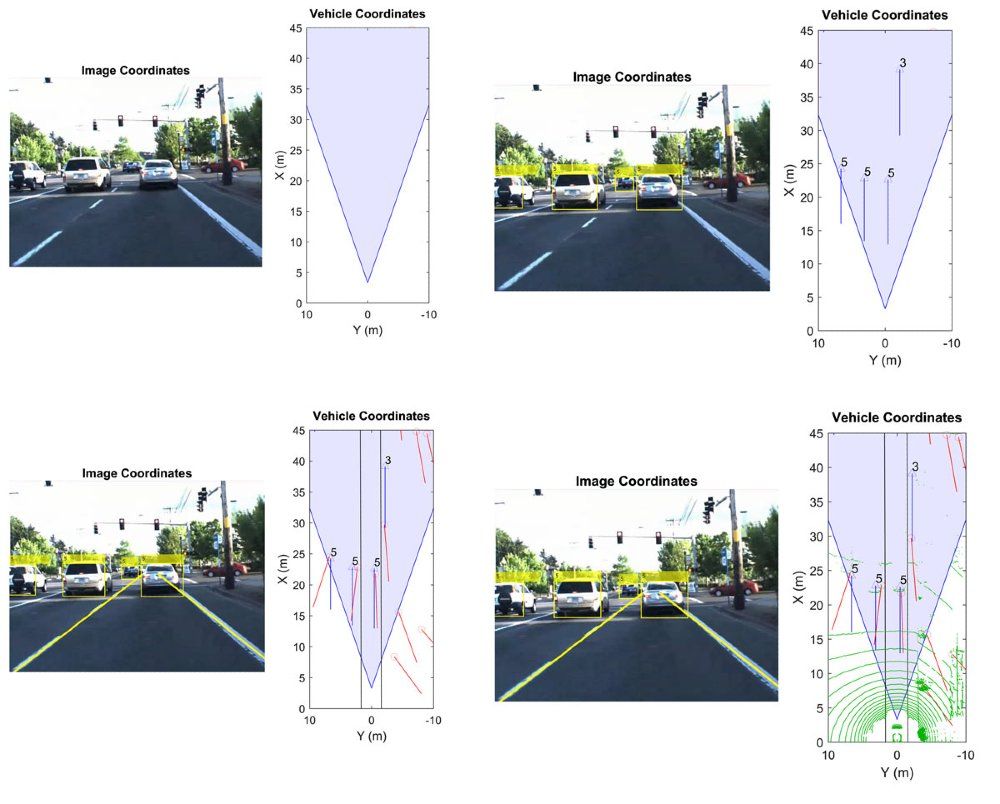This is a scientific diagram in a journal that consists of four quadrants, each displaying an image of traffic and a corresponding graph. The images show a scene from behind two or three cars stopped at a traffic light, each labeled at the top in black text with "image coordinates." The top left image is devoid of annotations, while the other three images (top right, bottom left, and bottom right) feature the same traffic scene with yellow and white boxes highlighting the vehicles.

Accompanying each image is a graph with a short y-axis and a tall x-axis, partially filled with a light purple triangle. These graphs provide detailed coordinates, with the y-axis labeled from 0 to 45 and the x-axis ranging from 10 to -10. In the graphs, the top right, bottom left, and bottom right quadrants include distinct lines and numbers, with the bottom right also containing green circles. The graphs appear to be mapping vehicle coordinates, as indicated by text such as "vehicle coordinates." Overall, this diagram meticulously illustrates how vehicle positions and movements are quantified and analyzed at an intersection, with a focus on detailed graphical representations.